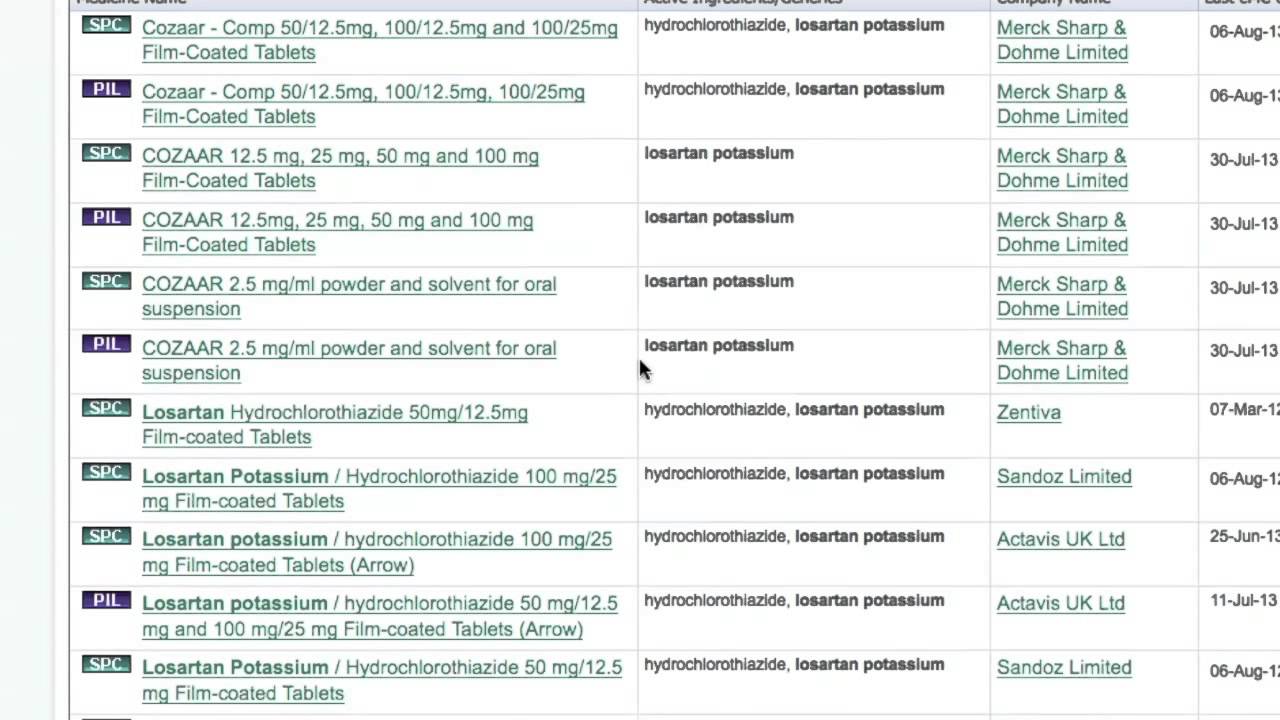**Detailed Caption:**

The image depicts a clean, white spreadsheet organized into five columns and eleven rows. The spreadsheet predominantly lists medications. The highlighted entries are for various dosages of Kosiar, which is written in green and includes the following dosages: 50/12.5 mg, 100/12.5 mg, and 100/25 mg, presented as film-coated tablets. Additionally, the spreadsheet lists hydrochlorothiazide alongside potassium, manufactured by Merck Sharp and Dohme Limited. The date August 6 is also present on the spreadsheet. The first seven rows of the spreadsheet indicate the same dosage for the listed medications, while the remaining four rows pertain to glossitarn potassium, with dosages of 12.5 mg, 25 mg, 50 mg, and 100 mg, also in film-coated form. No additional information is provided beyond these details.